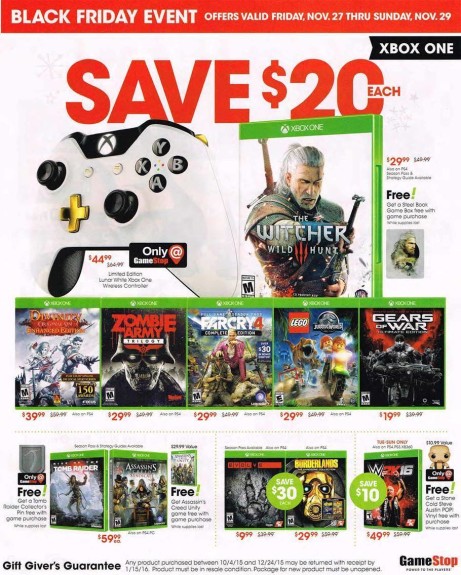The image depicts a promotional poster from GameStop, styled similarly to a magazine cover, advertising their Black Friday event. The main background is white, providing a clean and crisp canvas for the various game covers and details displayed. At the top of the poster, there's a red strip announcing the "Black Friday Event," specifying that offers are valid from Friday, November 27th to Sunday, November 29th. 

Prominently featured are several video games on sale, including "The Witcher 3," "Far Cry 4," "Gears of War," and a Lego-themed game, each bordered in green, indicative of Xbox One cases. Additionally, there is a spotlight on a discounted Xbox One controller, originally priced at $65, now available for $45—a $20 savings.

Across the bottom of the poster, there's a guarantee about the return policy, emphasizing customer satisfaction. The poster also highlights the GameStop slogans "Power to the Players" and "Gift to Givers," reinforcing the retailer’s commitment to providing great deals. The branding "Bonerize's GameStop" hints at a particular store or franchisee's personal touch on the advertisement.